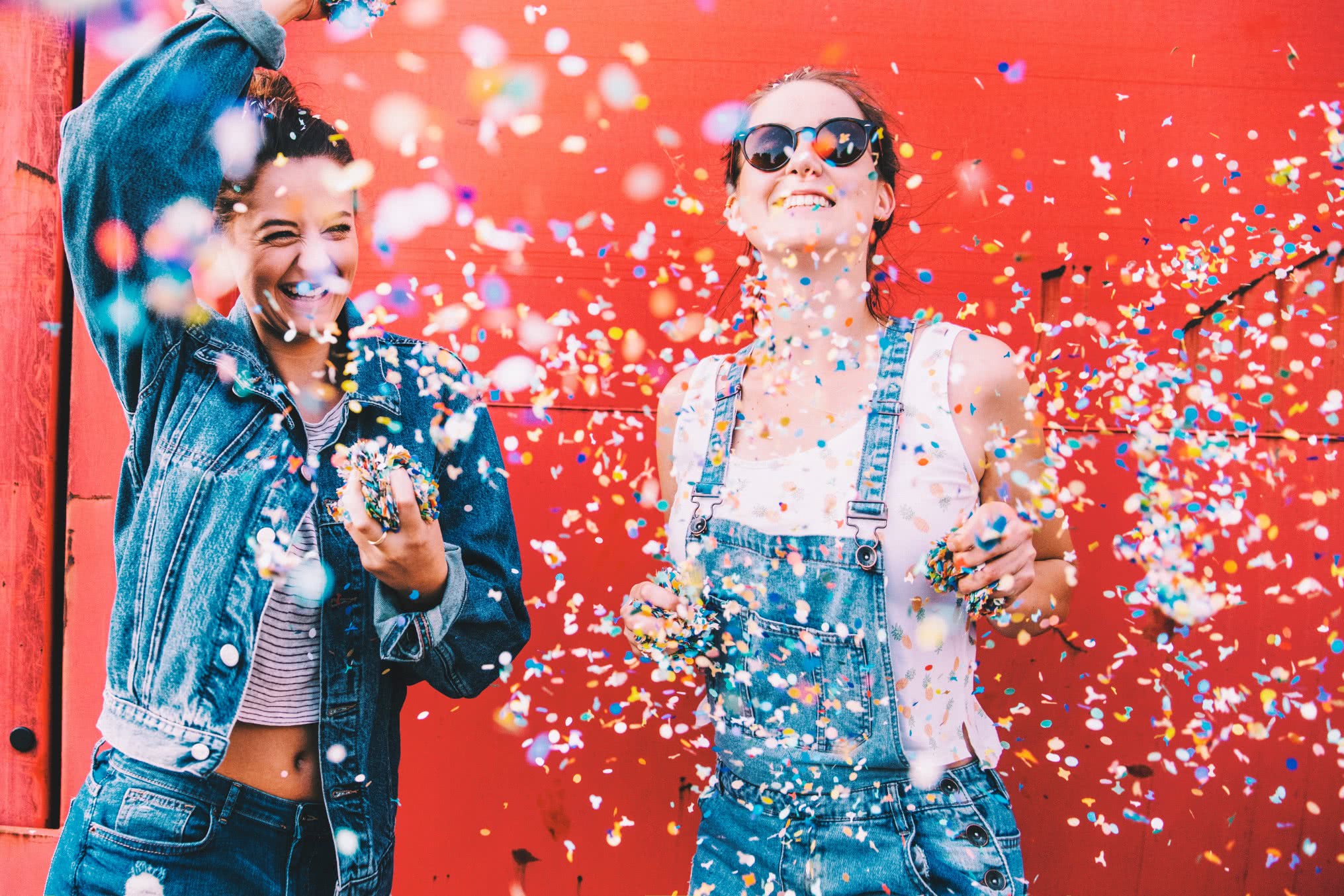In this vibrant outdoor image, a bright orange to red painted wooden wall forms the backdrop, featuring a vertical piece likely marking the edge of a windowsill on the left. In front of this striking background, two young, beautiful Caucasian women, both with darker hair and radiant smiles, are captured in a moment of shared joy. The woman on the left, dressed in a denim jacket, striped tank top, and jeans, showcases her midriff and holds a large ball of colorful confetti in her left hand. The woman on the right is adorned in denim overalls paired with a sleeveless white tank top and black sunglasses, clutching a sparkling ball of confetti in each hand. Confetti of various hues, including white, blue, and yellow, is scattered in the air, adding a festive and dynamic feel to the scene. Both women are animatedly engaged with the confetti, laughing and smiling, embodying a sense of fun and celebration.